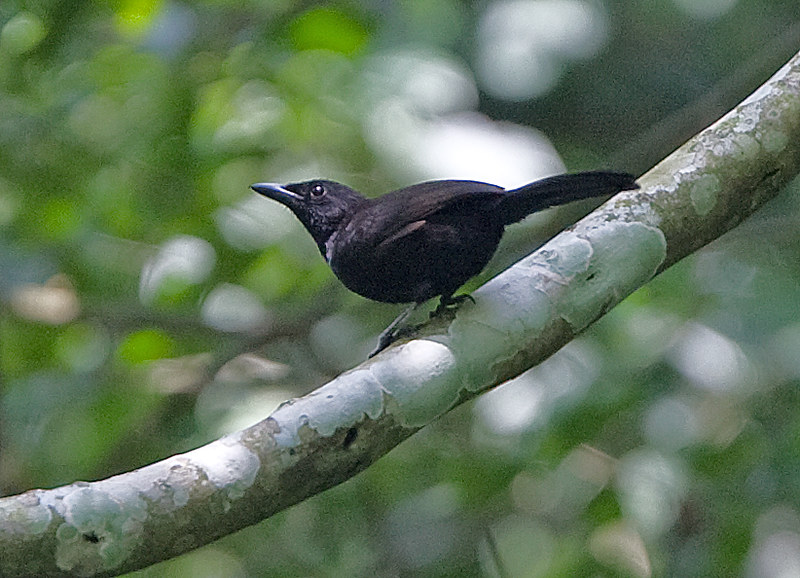The photograph captures a close-up view of a small bird perched on a weathered tree branch. The bird, about smaller than a robin, features striking dark plumage with a purple, brownish-black hue. Its glossy black beak and dark eye stand out prominently. The bird is hunched down, appearing as though it might take flight at any moment, with its wings pressed flat against its body and an impressive, albeit not overly long, tail extending several inches behind it. The branch it grips, roughly two inches in width, is silvery-gray and marked with greenish-gray patches, suggestive of moss or tree disease. The background, blurred to emphasize the bird and branch, hints at a forested setting with dappled shades of green and white, evoking a serene, natural environment.